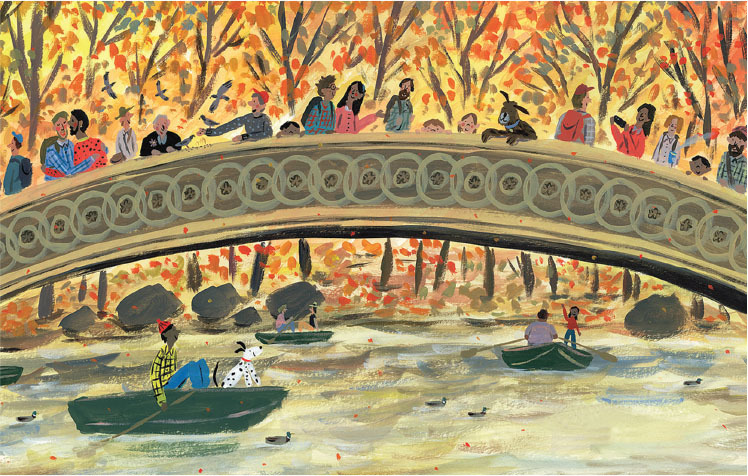This vibrant oil painting depicts a lively, joyful scene of diverse people and animals on an arched bridge over a serene river. The bridge, characterized by a circular patterned railing, is populated with a variety of individuals—different races, genders, and even a multiracial gay couple embracing on the left. Everyone is smiling, creating a sense of unity and happiness. There are people with backpacks, children peering over the railing, and a playful dog standing up and leaning over. Below, the river is dotted with ducks and three greenish boats. The foreground boat features a man in a yellow and black plaid shirt, blue pants, and a red hat, accompanied by a white and black Dalmatian. The backdrop of the painting showcases autumnal trees with vivid red, orange, and yellow leaves, enhancing the scene's warmth and charm. The attention to the varied yet harmonious details emphasizes the painting's simple, almost storybook quality.